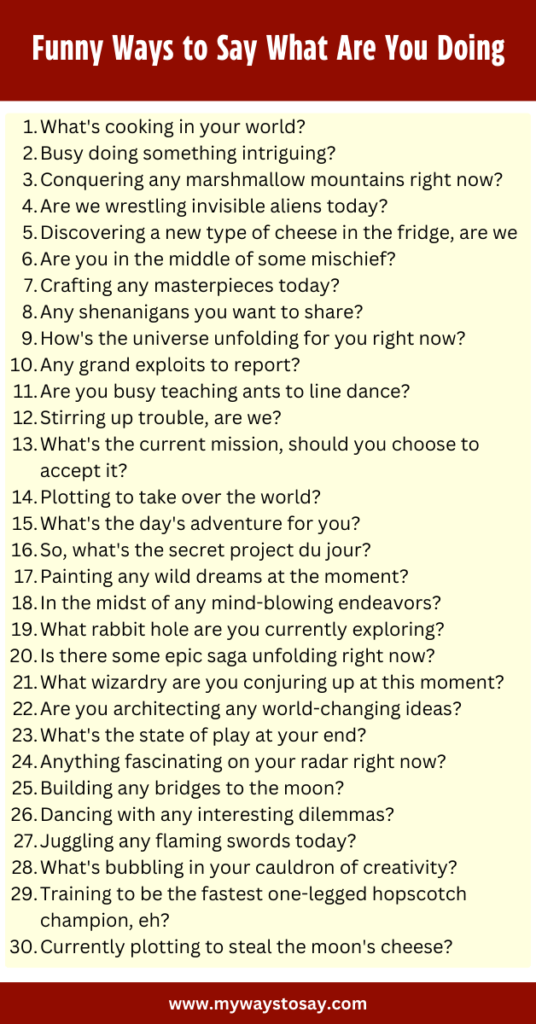**Caption: "30 Amusing Ways to Ask 'What Are You Doing?' - A Lively and Colorful Guide"**

At the top of the image, a bold red rectangle with white text serves as the title banner, reading "Funny Ways to Say 'What Are You Doing?'" Below this, a vibrant yellow background sets the stage for a list of 30 playful and humorous prompts, each numbered in black. Here's a closer look at the entertaining queries:

1. What's cooking in your world?
2. Busy doing something intriguing?
3. Conquering any marshmallow mountains right now?
4. Are we wrestling invisible aliens today?
5. Discovering a new type of cheese in the fridge, are we?
6. Are you in the middle of some mischief?
7. Crafting any masterpieces today?
8. Any shenanigans you want to share?
9. How's the universe unfolding for you right now?
10. Any grand exploits to report?
11. Are you busy teaching ants to line dance?
12. Serving up trouble, are we?
13. What's the current mission, should you choose to accept it?
14. Planning to take over the world?
15. What's today's adventure for you?
16. So, what's the secret project, dojo?
17. Painting any wild dreams at the moment?
18. In the midst of mind-blowing endeavors?
19. What rabbit hole are you currently exploring?
20. Is there an epic saga unfolding right now?
21. What wizardry are you conjuring up at the moment?
22. Are you architecting any world-changing ideas?
23. What's the state of play with you?
24. Any fascinating finds on your radar right now?
25. Building any bridges to the moon?
26. Dealing with any interesting dilemmas?
27. Juggling any flaming swords today?
28. What's bubbling in your cauldron of creativity?
29. Training to be the fastest one-legged hop-scotch champion?
30. Currently plotting to steal the most cheese?

This whimsical and detailed list is designed to inject some fun into the everyday question of "What are you doing?" by offering a variety of creative and amusing alternatives.